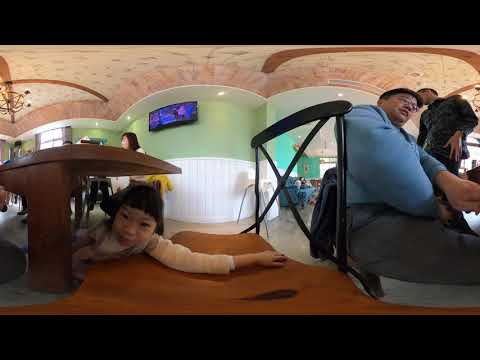The fisheye lens image depicts a somewhat distorted scene inside a spacious building, possibly a restaurant or public space like an airport or mall. Dominating the foreground, an Asian girl with a pageboy haircut lies on a brown carpet under a brown table, staring directly into the camera. She is wearing a white long-sleeve shirt, and her left arm is stretched out. An older Asian gentleman sits near the center-right, wearing a light blue top, gray pants, and glasses, looking downwards. Positioned behind him to the right, a young man with dark hair wears a gray and white long-sleeved jacket. 

In the background, walls painted light green on top and white on the bottom frame the scene, with a wide-mounted LED television displaying images, possibly of a sky and a tower. A conspicuous brown chandelier hangs from an arched ceiling above. Another woman with dark hair is barely visible above the table near the center-left, appearing to look left, and a masked young lady can be seen in the middle left section of the image. Light filters into the space, flooding the area around the patrons, highlighting the communal and bustling atmosphere of the venue.